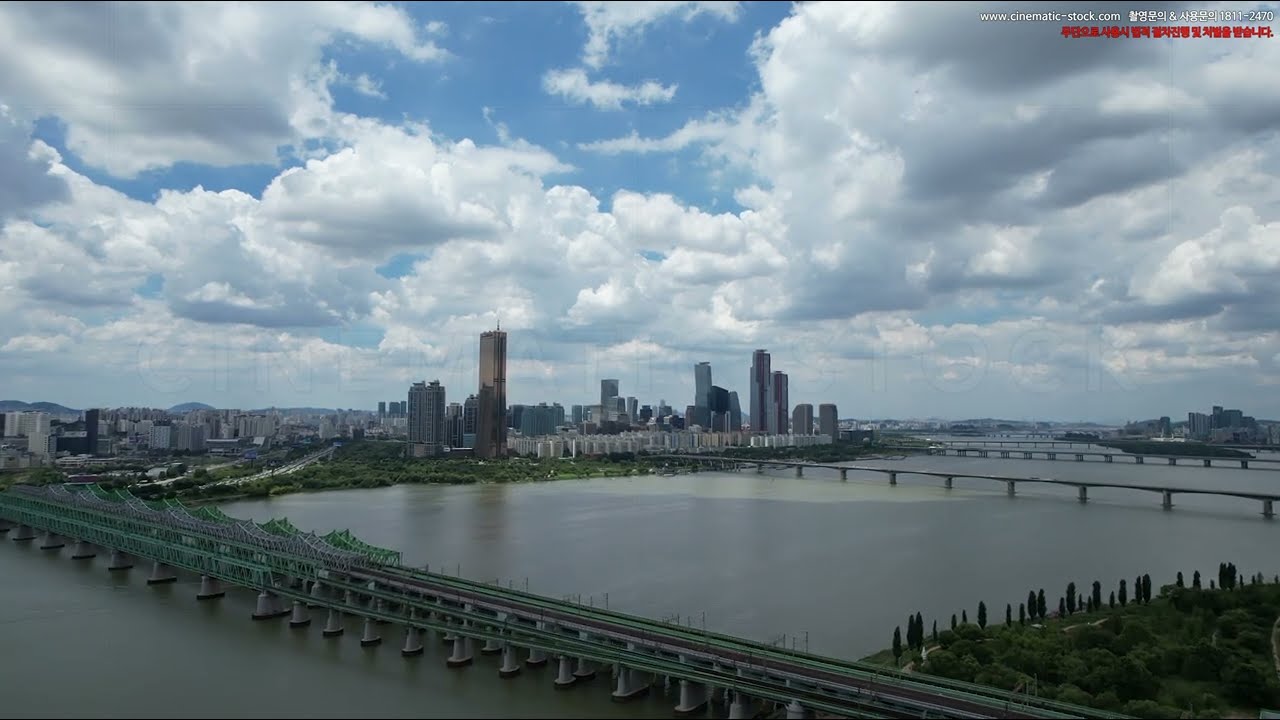This rectangular photograph captures a sprawling urban landscape beyond a large, somewhat uninviting gray-green body of water. A series of flat, low bridges span the water, supported by concrete pillars. These bridges vary in design, with the ones further back appearing more basic, possibly meant for trains, and the one closest to the viewer being a multi-level bridge for vehicles, adorned with typical metal grids and structures. In the foreground, a patch of land to the right is lush with green trees and grass. The far shoreline across the water is similarly green, dotted with areas of trees and shrubs before giving way to a dense cityscape. The city is characterized by a mix of skyscrapers and shorter buildings, with distinctive features like a copper-colored building near the water. The sky above is a light blue, filled with puffy white and light gray clouds, reminiscent of a "Toy Story" sky. Adding to the image, in the upper right corner, is text that includes a web address—www.cinematic-stock.com—accompanied by white and red Korean characters, with another set of red Korean characters at the bottom.